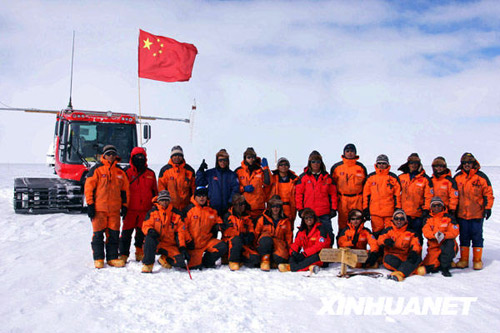The image depicts a large group of Chinese individuals in a snowy, polar region, possibly Antarctica or the Arctic. They are arranged in two rows, with the first row kneeling or sitting and the second row standing. Most of the people are wearing thick, bright orange jackets with either black or orange and black pants, although some in the group are wearing different colors; notably, one individual in the back row is in blue, and three others—two in the back row and one in the front—are in red jackets. Many of them have on hats and sunglasses. 

Behind the group, there is a substantial red vehicle with thick wheels, possibly a construction or expedition truck, equipped with a rectangular window and two protruding beams or antennas. Also at the rear is a Chinese flag flapping in the wind. The sky is clear with no clouds visible, adding to the bright and sharp clarity of the photograph. At the bottom right corner of the image, in white, slightly faded text, the word "XINHUANET" is written in capital letters. The overall scene conveys a sense of teamwork and expedition under harsh, snowy conditions.